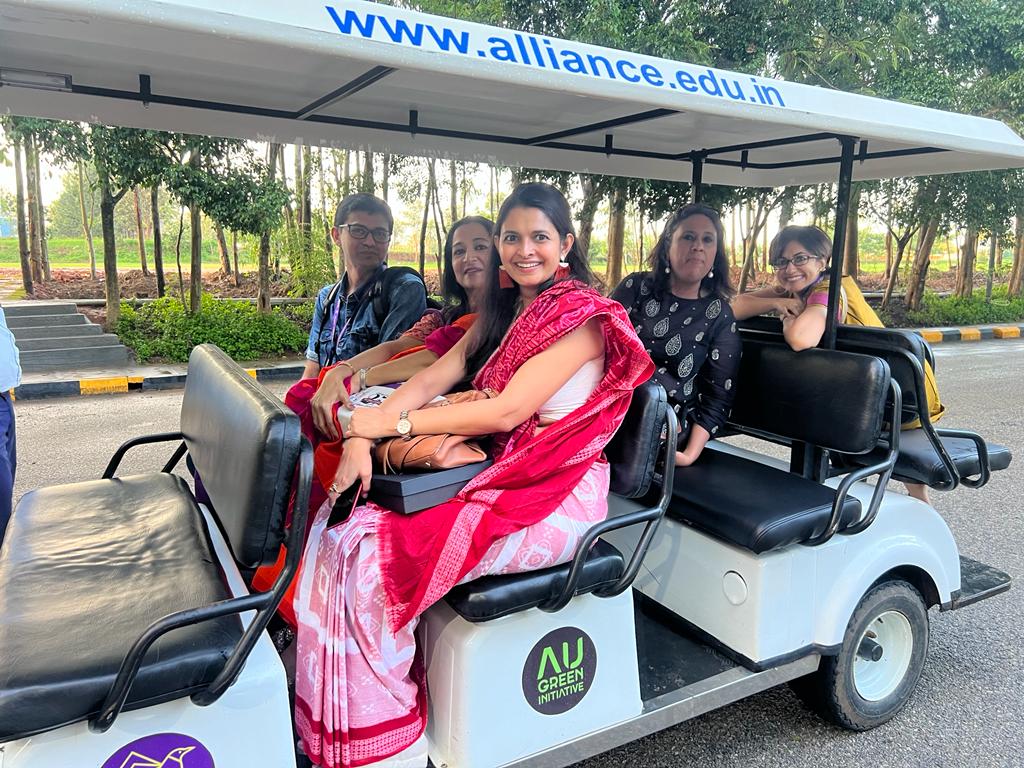The landscape-oriented image captures a white golf cart with four rows of black cushioned seats. The first row on the left is empty, while the second row seats three people—two women and a man—dressed in traditional, bright Indian attire. The third row holds a single woman, and the final row faces backward, with one woman turning around to smile for the photograph. The golf cart features a roof with blue text that reads www.alliance.edu.in. A purple and yellow logo is visible below the seat of the first row, and another black and green logo is under the second row, indicating "AU Green Initiative." In the background, there is an asphalt road bordered by trees and a curb, creating a verdant, relaxed setting.